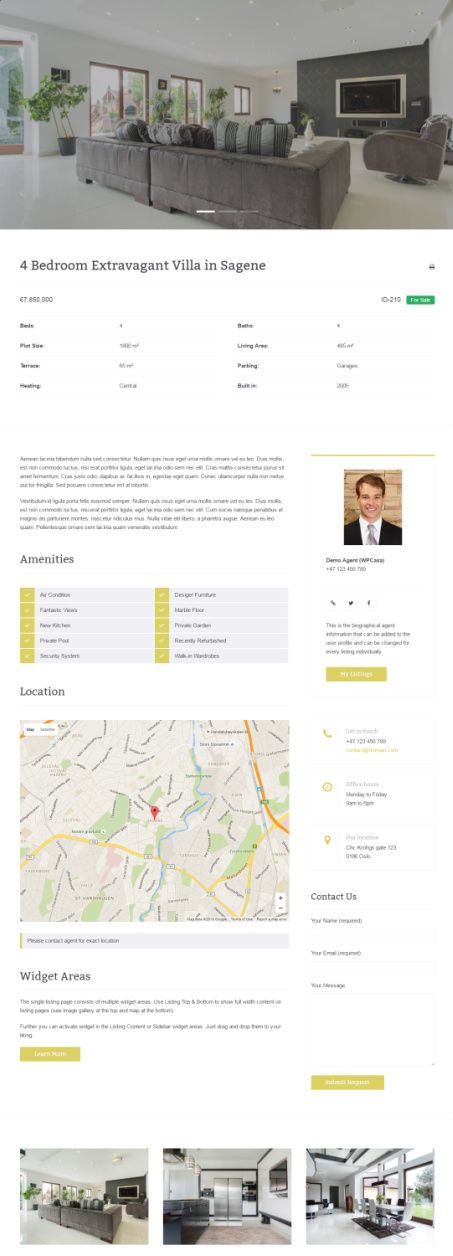The image features a detailed promotional graphic set against a white background. At the center is a photograph of a luxurious villa, labeled "Four Bedroom Extravagant Vow and Villa." Although the text on the house image is largely illegible, it appears to say "SAGENE" or "EVEZE." To the right of the image, there are four informational columns.

The top section includes two rectangles - one white and one green - containing various pieces of information. Below this, a professional portrait of a man dressed in a black suit with a white collared shirt and a red and blue tie is displayed. Accompanying the portrait is detailed information about the man's credentials and expertise.

The amenities offered by the villa are outlined in a chart format nearby. Next to this is a map pinpointing a specific location, indicated by a map logo. Also visible are contact details presented in a structured layout, which include a phone icon with a phone number and an address with a location logo. Additionally, there appears to be an area dedicated to contacting the establishment, featuring interactive widgets for user engagement.